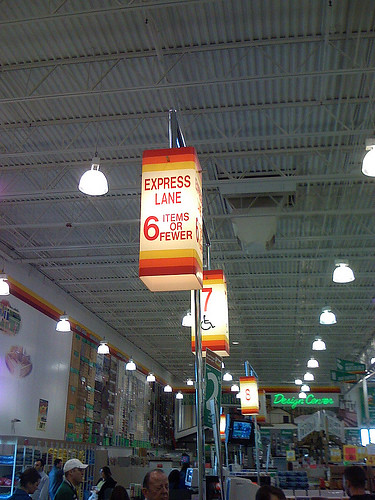In this vibrant color photograph taken inside a bustling store, the shot captures several lanes leading to different cash registers. The lane in the foreground is marked with a sign overhead that reads "Express Lane, six items or fewer." Just beyond it, another lane is labeled with a number seven and features a handicapped symbol, indicating accessibility for individuals in wheelchairs. Further still is lane eight, distinguishable by its simple numeric sign. In the background, a glowing green neon sign proudly announces the "Design Center." The ceiling of the store reveals an industrial style, characterized by exposed ductwork and numerous white lights that illuminate the space. Items hang on the walls, though they are not clearly visible in the image. In the bottom left corner, a crowd of people can be seen milling about, adding to the lively atmosphere of the scene.